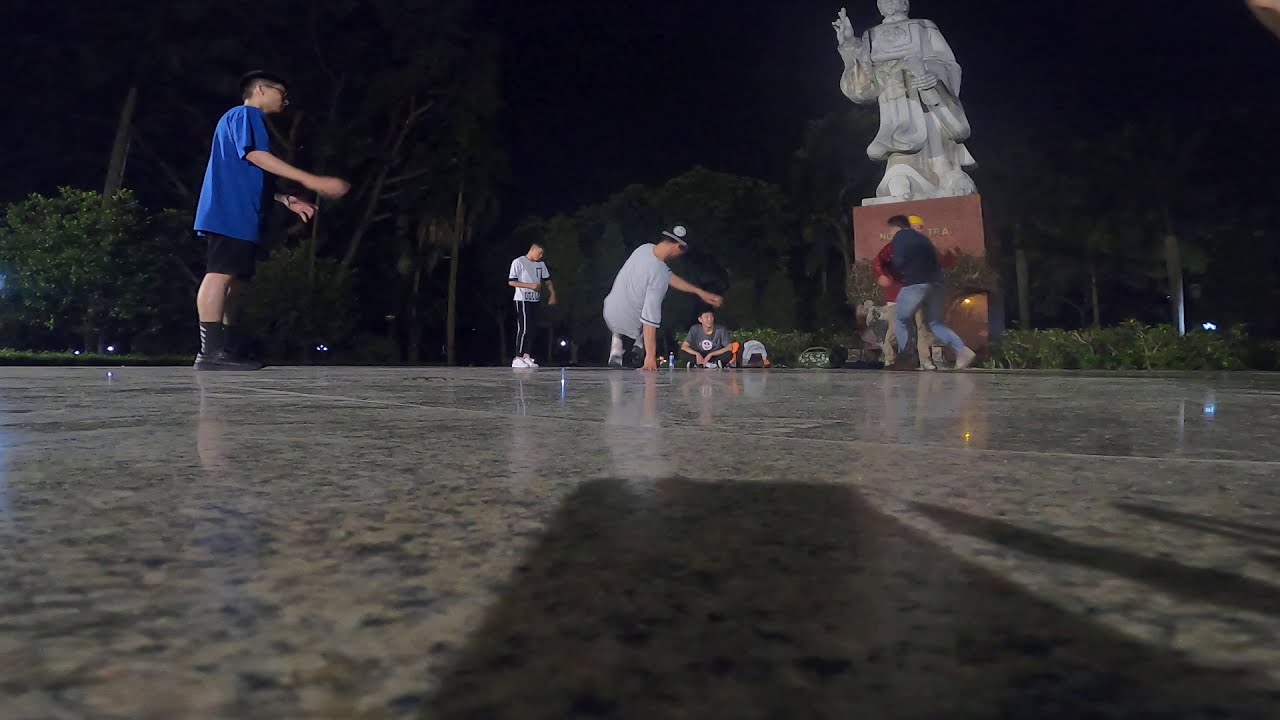The nighttime image captures a vibrant scene in an outdoor park with a glossy stone surface, likely marble or granite. The camera perspective is low, offering an eye-level view of a group of breakdancers approximately 10 to 15 feet away. At the center of attention is a large stone statue on a pedestal, depicting a man in a robe with one hand raised, standing about 15 to 20 feet tall. The background is filled with tall green trees and shrubs.

In front of the statue, a dynamic breakdancing session unfolds. A performer in a gray shirt, white tennis shoes, and a backwards black hat is captured mid-move, balancing on his right hand. Surrounding him in a loose half-circle, five other dancers and bystanders are dressed in casual athletic wear, including an Asian man on the left in a blue t-shirt and black shorts. Additionally, two people near the statue seem to be embracing, while another is running or possibly joining the dance. The entire scene is imbued with an energetic, communal atmosphere, set against the dramatic backdrop of the dark night sky.